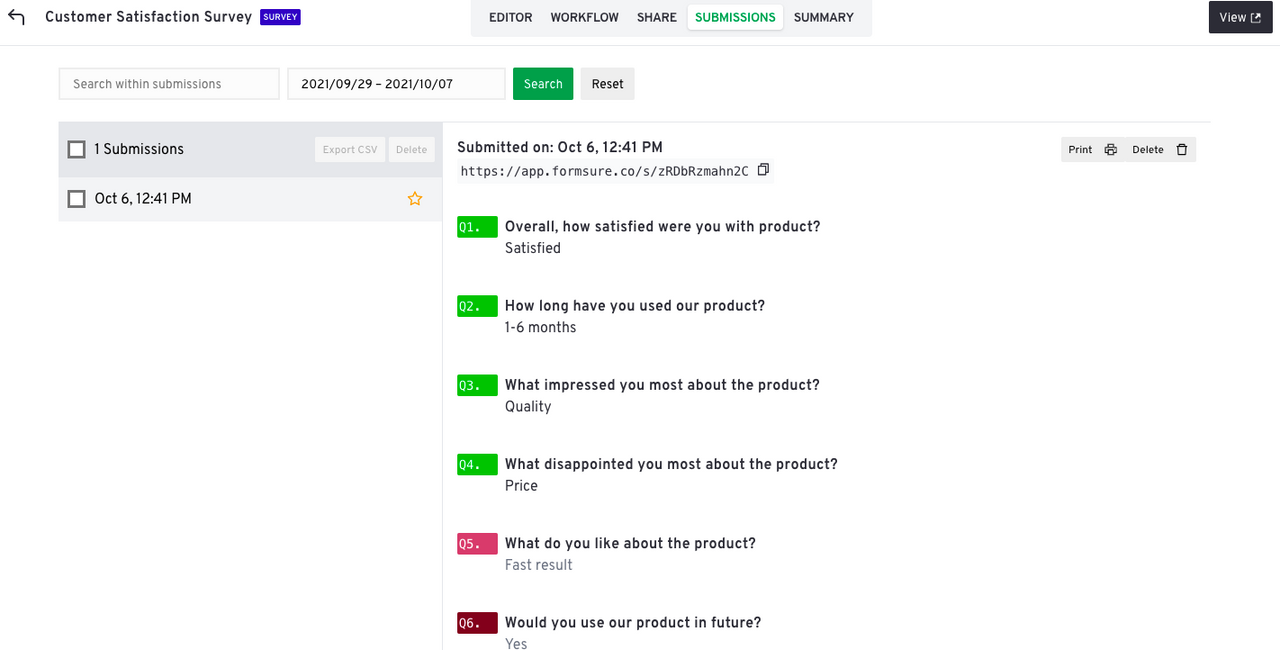**Detailed Caption:**

The image is a screenshot from a website reflecting a customer satisfaction survey. In the top-left corner, the text "Customer Satisfaction Survey" is prominently displayed, accompanied by a small, purple-grey rectangular tab with the word "Survey" written in white.

Centrally placed is a light grey navigation bar containing five options: Editor, Workflow, Share, Submissions, and Summary. The option "Submissions" is highlighted in green, differentiating it from the other options which are displayed in black.

Below the navigation bar, the survey details are presented. The text reads: "Submitted on October 6th, 12:41 PM." The survey questions and their respective responses are listed as follows:

1. **Overall, how satisfied were you with the product?**
   - Answer: Satisfied
  
2. **How long have you used our product?**
   - Answer: 1-6 months
   
3. **What impressed you most about the product?**
   - Answer: Quality
   
4. **What disappointed you most about the product?**
   - Answer: Price
   
5. **What do you like about the product?**
   - Answer: Fast results
   
6. **Would you use our product in future?**
   - Answer: Yes

Next to questions 1-4, there are green rectangles serving as markers, while question 5 has a pink rectangle and question 6 has a wine-colored one. The structured layout and use of colors effectively differentiate each section of the survey, making the information clear and accessible.